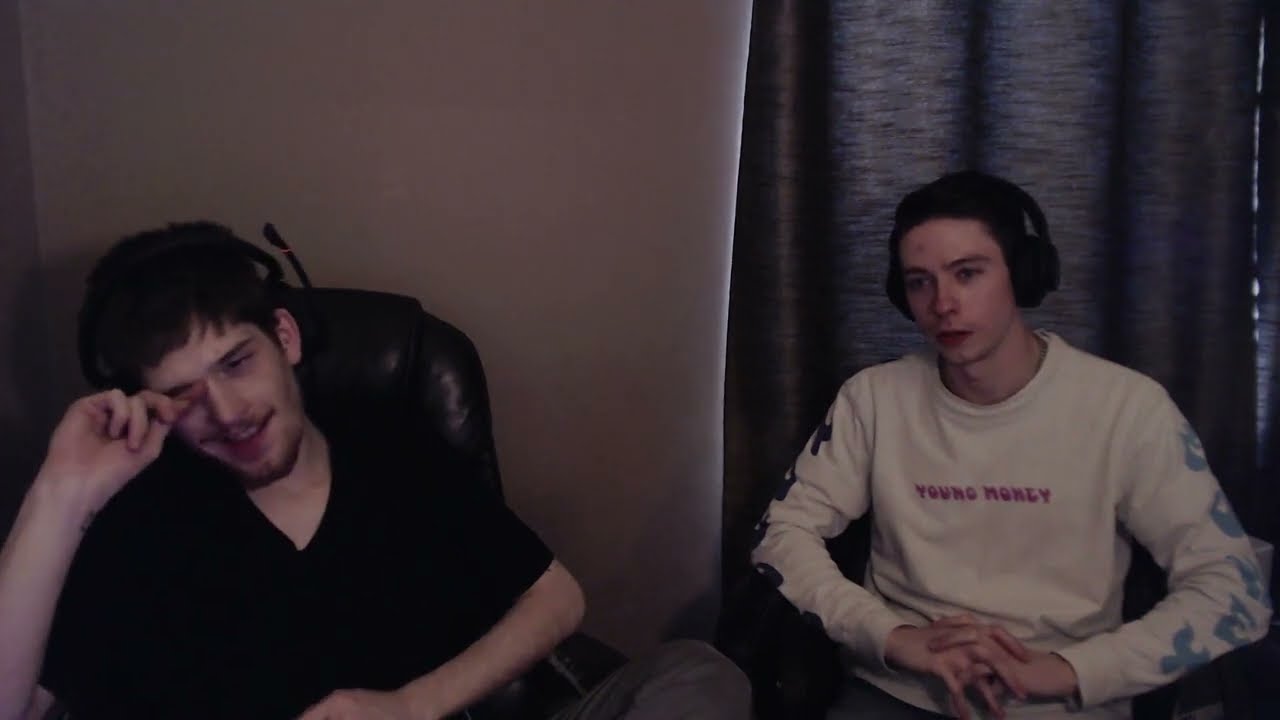The image features two young men, likely around 19 or 20 years old, seated next to each other. Both are wearing headsets, suggesting they might be playing a video game together. The man on the left, with long brown hair, a mustache, and a slight beard, is dressed in a black V-neck t-shirt with short sleeves. He is seated in a brown leather chair and is covering his right eye with his right hand, as if rubbing it. His headset includes a microphone positioned on the left side of his head. 

The man on the right, who is light-skinned and clean-shaven, is wearing a white long-sleeve t-shirt with red "Young Money" lettering on the front. The sleeves of his shirt have distinct patterns, with a light blue design on his left arm and a black design on his right arm. He is seated in front of a dark blue curtain, which partially reveals a window as light seeps around it. His hands are crossed in front of him, with fingers interlaced.